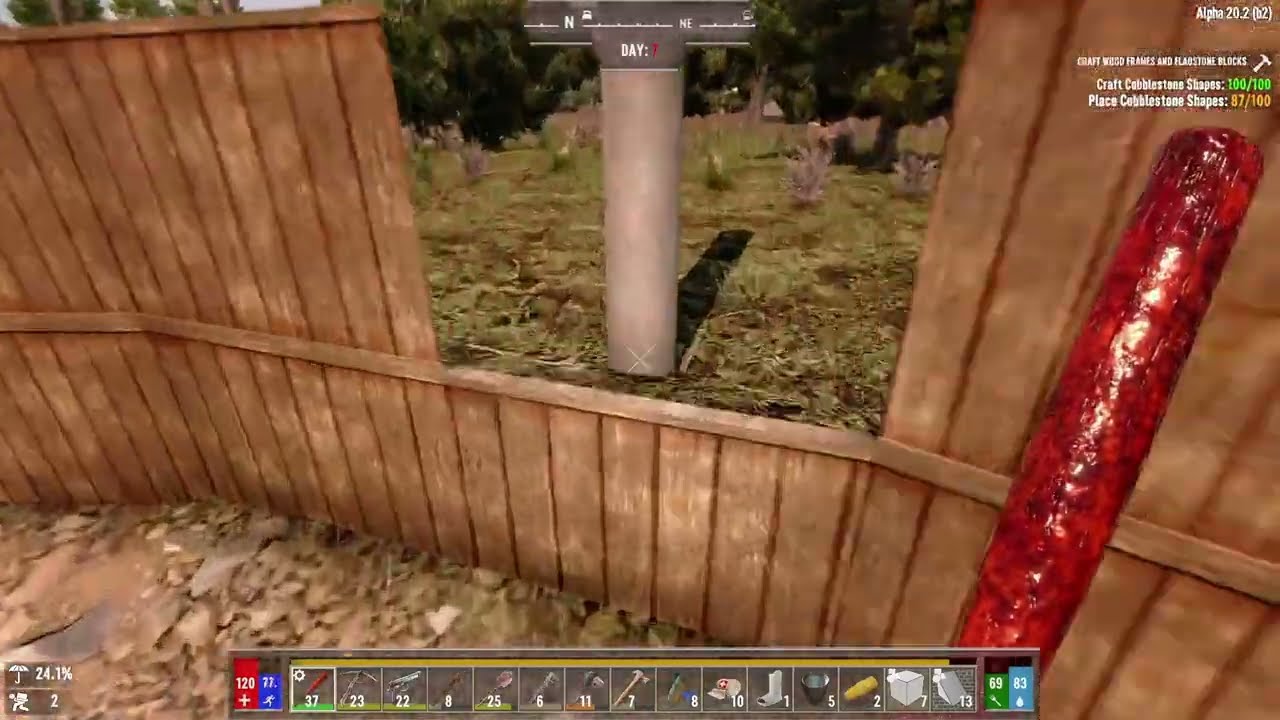The image appears to be a screenshot from a video game, prominently featuring a detailed wooden brown fence with both vertical slats and horizontal pieces. In the center of the fence, there is a cutout resembling a window, through which green grass and a tall gray column are visible. Above the fence, the tops of green trees or bushes can be seen. 

To the left of the window in the fence, brown dirt and light brown mulch are present. The bottom tray of the screen contains various numbered squares, including the sequence: 37, 23, 22, 8, 25, 6, 11, 7, 8, 10, 1, 5, 2, 7, and 13. In the bottom left corner of the screen, an umbrella icon displays "24.1%", accompanied by a person icon with the number 2 beneath it.

Towards the top of the screen, there is a compass indicator and text reading "Day 7". In the upper right corner, white text displays "Alpha 20.2 B2" and "place cobblestone shapes 87/100". The player is holding a brownish-red cylindrical object seen on the right side of the image.